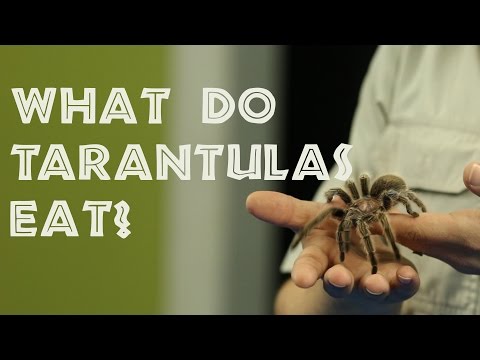The image is a rectangular PowerPoint presentation slide featuring a central photograph of a man holding a live tarantula. The man, whose facial features are not visible, is wearing a beige or khaki pocketed zookeeper-style shirt, and stands indoors against a backdrop that includes a bright green wall with white trim around a doorway. The man is holding the large, brown, furry tarantula with both hands: his right hand is palm-up holding the tarantula, while his left hand supports the spider’s left legs. The tarantula appears sizable, filling the palm of his right hand. The top and bottom of the image are bordered with medium-thick black bands. Overlaying the photograph, in large, all-capital white text, is the question “WHAT DO TARANTULAS EAT?”.